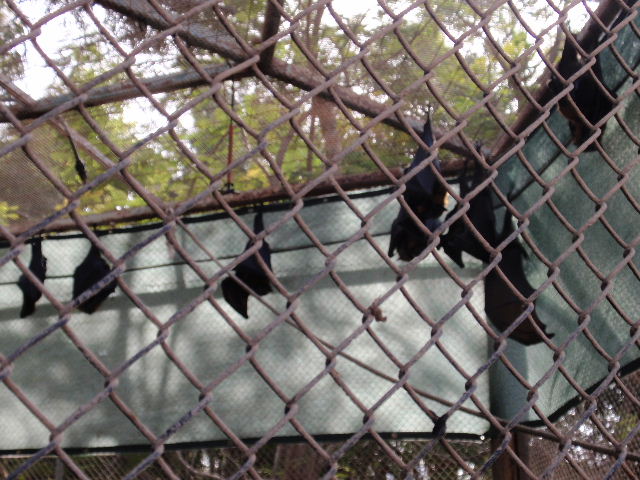This color photograph captures a bat enclosure cage from an outside perspective. The cage is predominantly constructed from rusted chain-link fencing, which lines the top, bottom, and sides. Inside, seven dark, black-colored bats hang upside down, most with their wings tucked into their bodies, indicating they are sleeping. The roof of the cage features a green felt covering, likely to provide shade from the sun, and is supported by rusty beams forming a fork shape across the top. The enclosure is situated beneath a canopy of light green leaves from surrounding trees, clearly visible in the upper portion of the image. The photograph, taken during the day, reveals these details through the square openings of the fence, with some bats appearing closer to the viewer and others slightly further away.